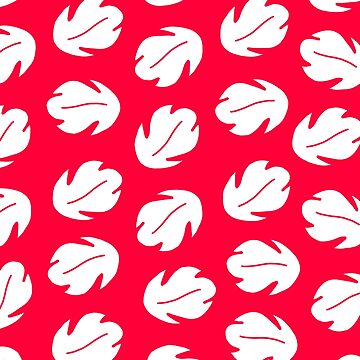The image features a bright red background adorned with a pattern of white leaves, which are simple in design and adorned with little curved points. The leaves are arranged in columns, with each column separated by a space of red background, creating a rhythmic pattern. These leaves have a central red vein that extends outward, giving them a distinctive look. They vary in their orientation, alternating diagonally in multiple directions, including diagonal right, diagonal left, and upward and downward angles. This layout forms a dynamic, eye-catching design that could be used as wrapping paper, wallpaper, or even patterned fabric. The repetitive and orderly arrangement of the leaves against the vibrant red backdrop creates a striking visual effect.